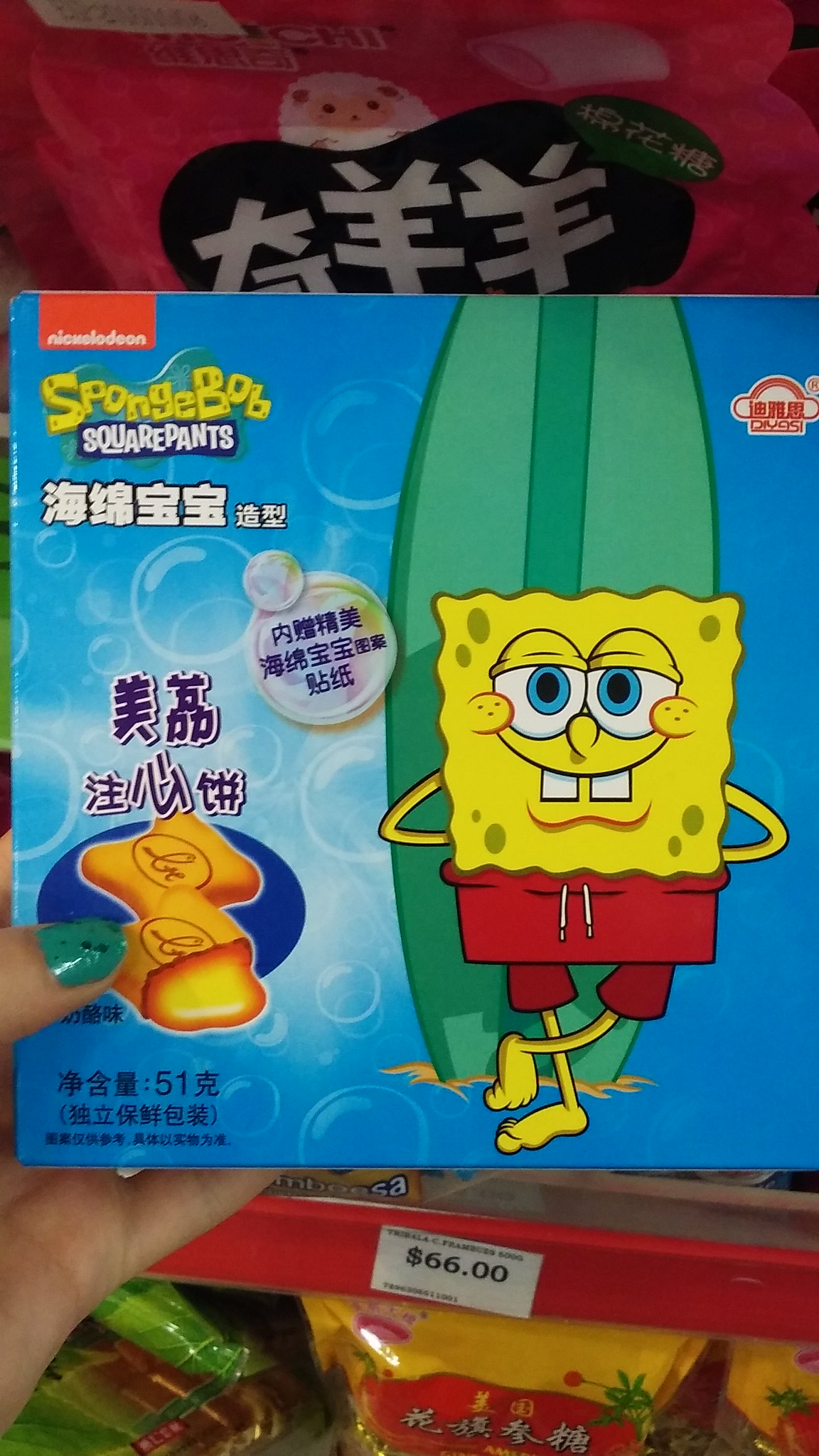This detailed color photograph showcases a packaged treat with a vibrant blue background. The rectangular package features the iconic character SpongeBob SquarePants, who is depicted with his characteristic yellow sponge face, big white eyes with blue pupils, and buck teeth. Intriguingly, SpongeBob sports red shorts and stands cheerfully next to a light green surfboard that has a dark green stripe running vertically down its center. Above SpongeBob, "Nickelodeon" is prominently displayed in white letters on a red background, and the rest of the package text is written in either Chinese or Japanese. A person's hand, adorned with painted fingernails, holds up the package revealing shelves below filled with various plastic-wrapped snacks, as well as another bag with oriental writing partially visible. The edible product itself, slightly opened at one end, shows a tan to dark brown exterior with a creamy filling, adding a delectable touch to the visually engaging scene.